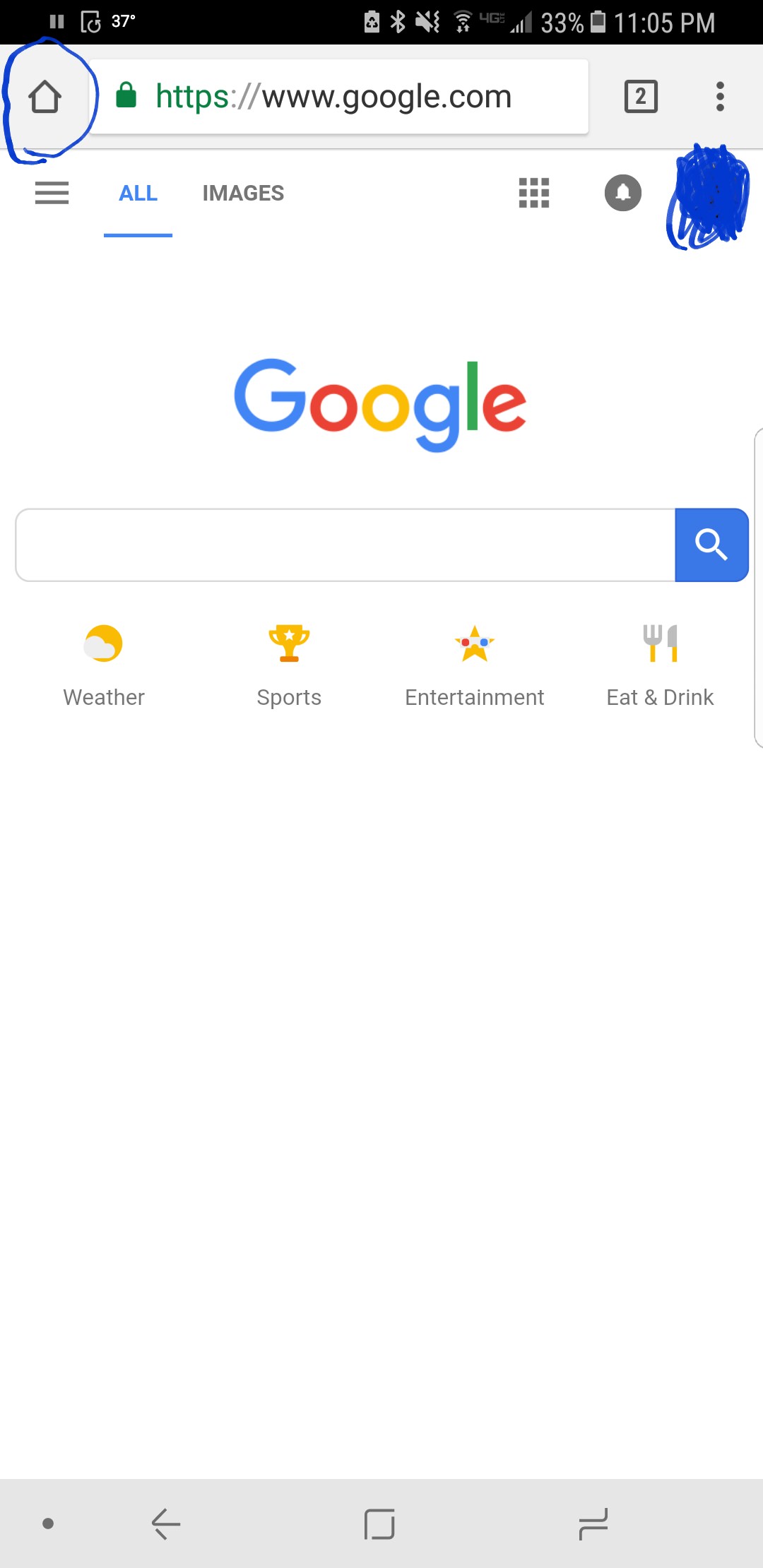The image is a portrait-mode screenshot taken from a cell phone. In the upper left-hand corner, the temperature is displayed as 37 degrees. The upper right-hand corner shows a battery level of 33% and the time, 11:05 p.m. Below this, there is a black stripe followed by a gray stripe. Next, there's a rough hand-drawn image of a house. Below, the URL "www.google.com" is visible in a search bar. To the right of the search bar, a square with the number "2" indicates that two tabs are open, followed by three vertical dots representing more options.

In the next section, two tabs are visible, labeled "All" and "Images." The "All" tab is highlighted in blue and underlined. On the right side, the user’s avatar is heavily scratched out in blue to maintain anonymity. The Google logo appears next, featuring its usual blue, red, yellow, blue, green, and red colors. Below the logo is another search bar. Four icons for "Weather," "Sports," "Entertainment," and "Eat and Drink" are situated directly beneath this search bar, each accompanied by a relevant picture.

The remainder of the screen is a large white space, leading down to a broad gray stripe at the bottom. This stripe contains four navigation icons: a dot, a back arrow, a square, and an icon with lines resembling an ascending and descending line meeting in the middle. Each Google icon has a matching image corresponding to its label.